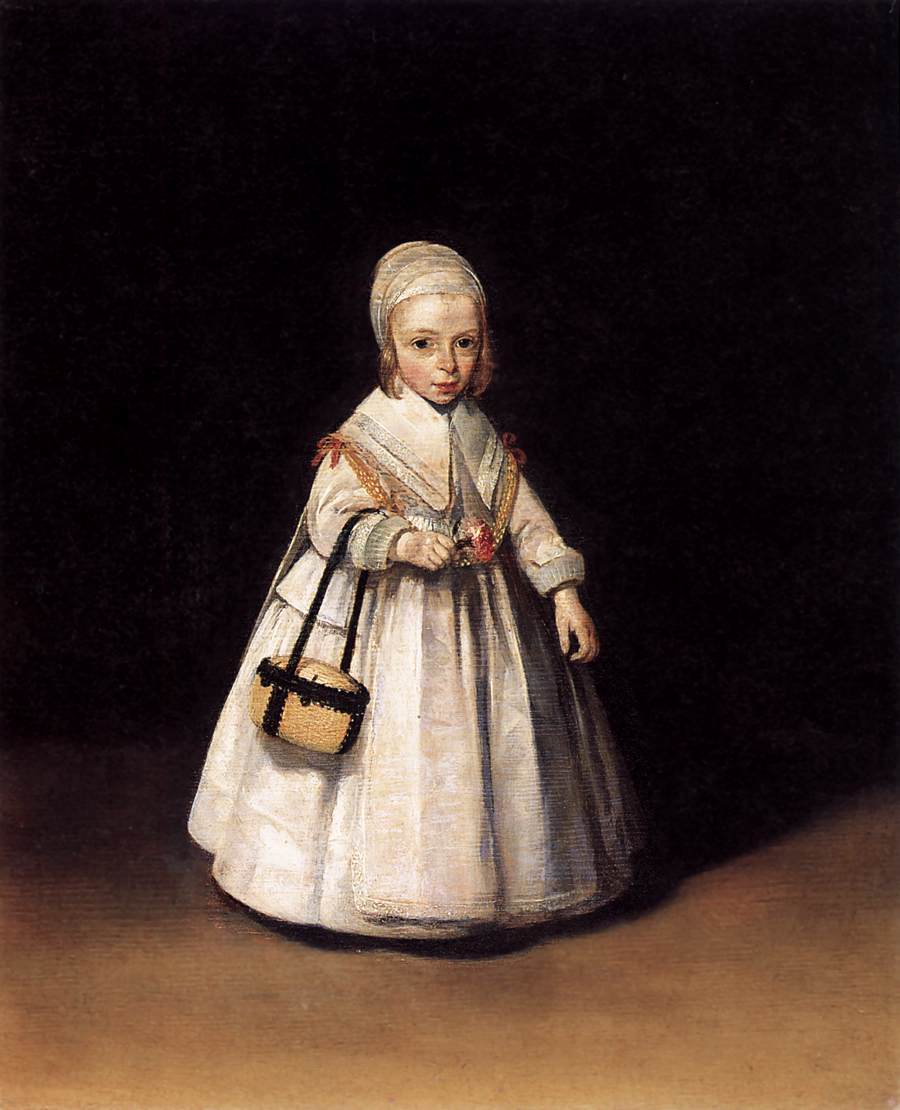The vertically aligned rectangular image presents an evocative, old-style painting dominated by a dark atmosphere. The top half is engulfed in a solid black background, which transitions into a darker brown in the middle, ultimately leading to a tan or brown flooring at the bottom. At the center stands a young girl, or possibly a small woman with features suggesting a potential disability, given her mature facial expressions yet small stature of around three feet. She dons a grayish-white, heavily pleated long dress that completely covers her feet, and a bonnet or headscarf with slight hints of blondish-brown hair peeking out from the sides. Her expressive big, dark brown eyes gaze directly at the viewer while her mouth remains closed. A shawl with golden-red trim is elegantly wrapped around her shoulders, over the thick cuffs of her sleeves. Her right arm, bent at the elbow, supports a tan and black bag or purse that could be handmade, evoking a rustic charm. The left arm hangs down naturally by her side. The overall scene exudes a deeply historic and somber ambiance, heightened by the strong contrast between the dark background and the brown flooring.